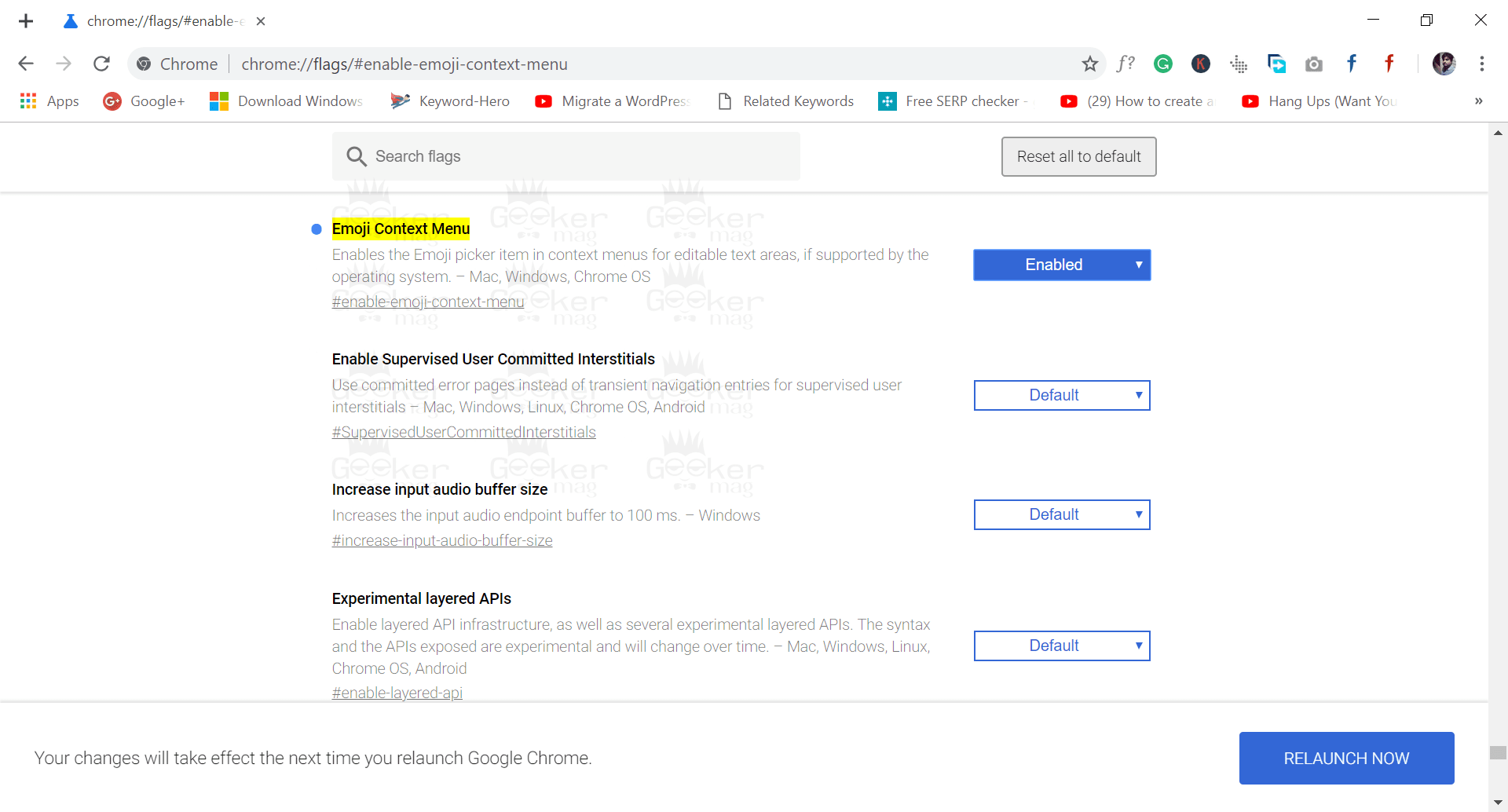This is a screenshot of the Chrome browser settings page, specifically displaying the "chrome://flags" section. The browser is in light mode, featuring a white background with black text. At the top, just beneath the URL bar, several tabs are pinned, signifying frequently visited sites. Directly below, there is a search bar placed within a light gray box, containing the placeholder text "Search flags." Adjacent to the search bar, there is another light gray box labeled "Reset all to default." 

The main content area is divided into sections, each representing different experimental features of the browser. Each section has various options, with their current status indicated by blue boxes. These boxes alternate between being positioned to the left and the right. The statuses visible in the screenshot include "Enabled," "Default," and "Disabled." Notably, the first three sections have blue boxes to the right labeled "Enabled" or "Default," while the fourth section features a blue box to the left marked "Disabled."